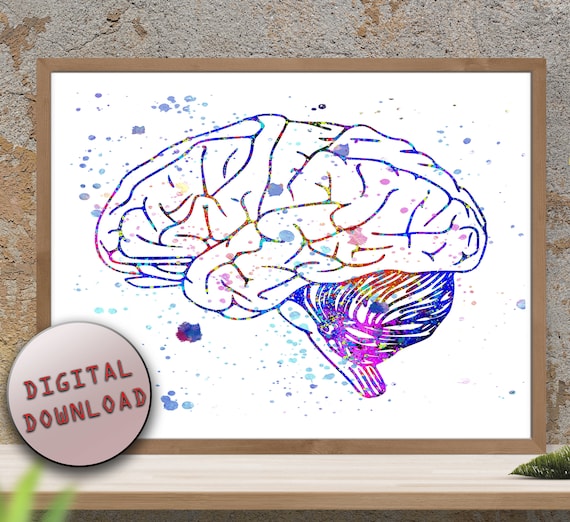This detailed caption combines the information provided, emphasizing shared observations and notable details:

The image showcases a framed illustration of a human brain, rendered in vibrant, rainbow-like colors that delineate its various sections. The artwork is propped up on a wooden mantel against a masonry-style, grayish-brown wall. The frame is thin and wooden, complementing the artwork within, which features a white background. Alongside the multicolored brain illustration, there are artistic splatters of blue and pink paint scattered throughout. Notably, in the bottom-left corner of the image, there is a circular icon with the words "digital download" in red font. The brain illustration also includes detailed line work, particularly in the area at the top of the spine, with shades of blue, pink, and red extending beneath the main structure. Additionally, some green plants can be seen at the bottom of the image, though they are out of focus.